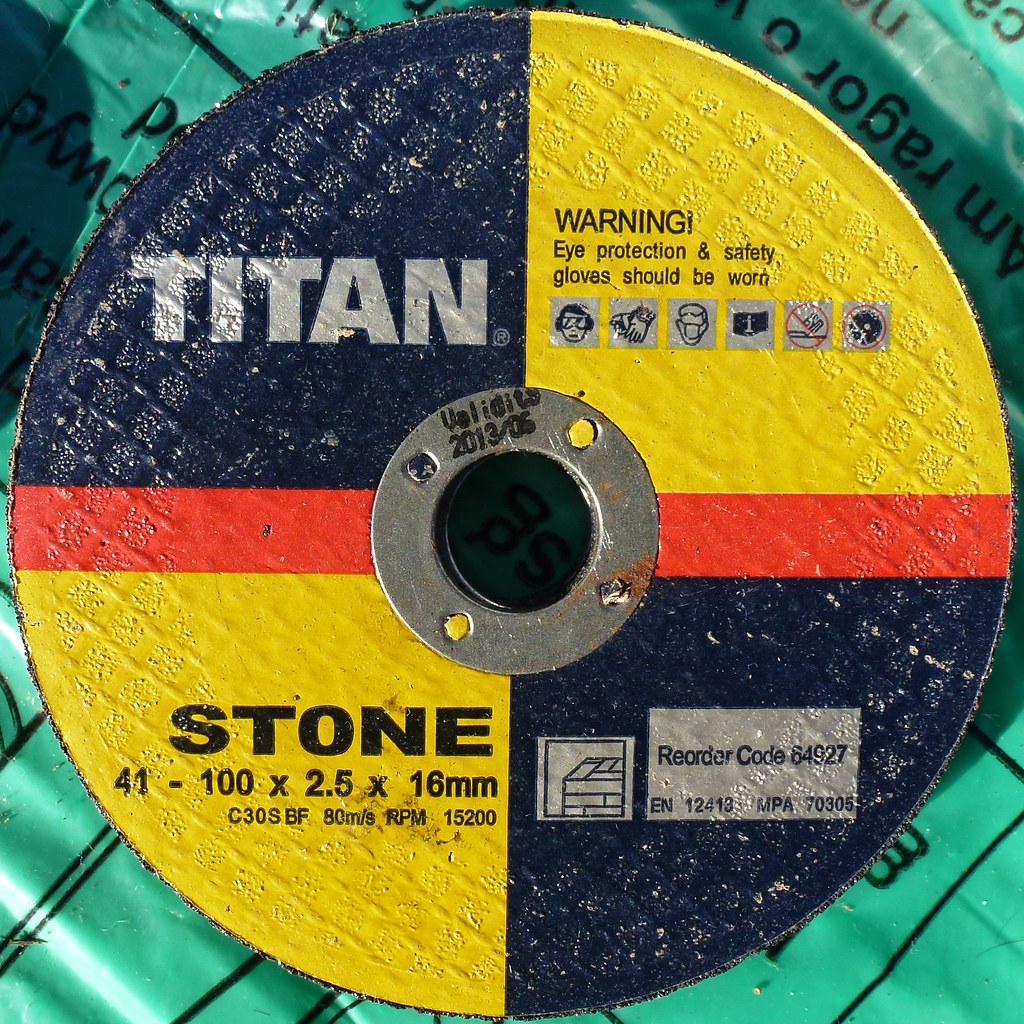The image prominently features a circular disc laying on a green plastic surface, likely at a construction site. The disc is segmented into four parts, resembling a nuclear symbol, with a distinct red stripe running through the middle. The top left section bears the word "Titan" in a white or light gray font set against a navy background. Adjacent to it on the top right, a yellow backdrop displays a warning: "Eye protection and safety gloves should be worn," accompanied by six small images, including depictions of glasses, gloves, a face mask, the letter 'I', and other safety-related icons. At the bottom left of the disc, text in black reads "Stone 41-100x2.5x16mm," and to the bottom right, a white box contains the reorder code "864927." The overall color palette includes black, green, yellow, red, dark blue, and gray, with the circular disc positioned centrally, taking up most of the image. The background setting appears to be outdoors, possibly highlighting a construction context.